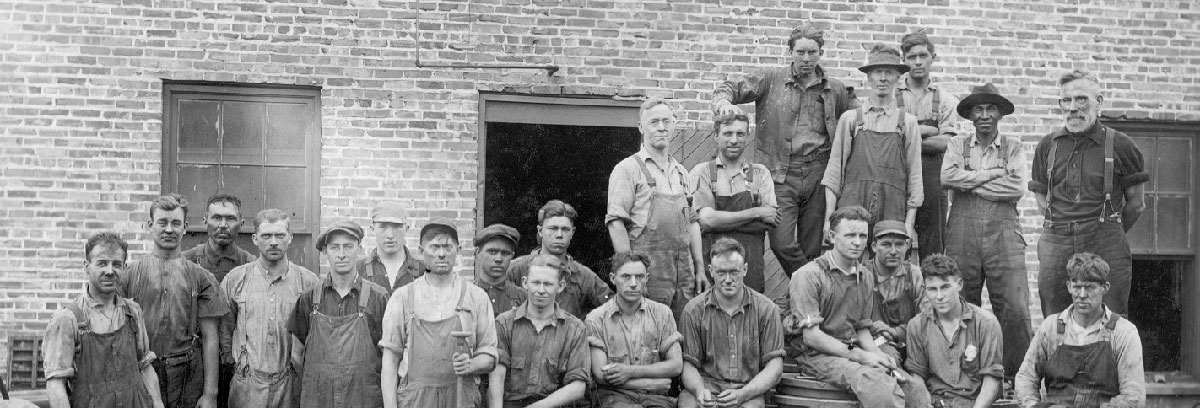In this old black-and-white photograph, a group of about 20-25 men is posing in front of a brick building, likely a factory. Most of the men are dressed in denim overalls and shirts with the sleeves rolled up to their elbows or biceps, indicative of manual labor. Their faces appear grimy, suggesting they have been hard at work, possibly in coal mining or another physically demanding job. Despite their rugged appearance, none of the men are smiling; instead, they squint at the camera, with a couple crossing their arms. Among the group, one older man stands out, dressed in darker clothes with suspenders and a dark shirt, and sporting a white beard, likely positioning him as a supervisor or boss. The men are arranged in two rows, with some standing on an elevated surface on the right side, making them appear taller against the kiln brick backdrop, which includes simple windows and an open door. The horizontal composition of the photograph, combined with the vintage attire and the lack of color, hints that this image was captured in the 1930s or 1940s.